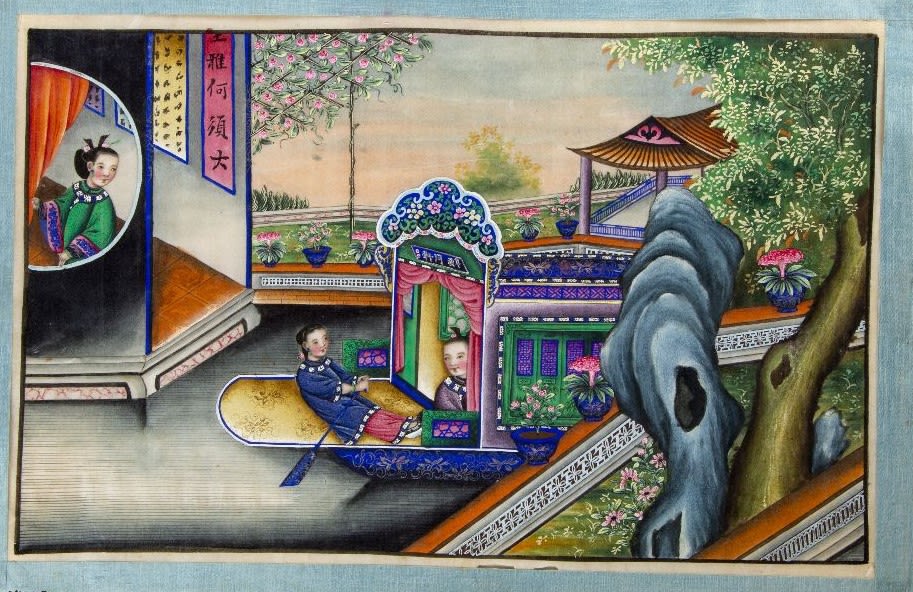This vibrant traditional painting, rendered in a pastel chalk style, is encased in a light blue rectangular frame with a white inner outline. The scene is divided into two main sections. On the left, there's a half-circle entrance leading into a Japanese-style room. Inside, a woman dressed in a green robe and with her hair styled traditionally gazes out of a window. Japanese text adorns the wall, and a red curtain adds a bold accent.

To the right of this room, a large, colorful garden unfolds. In the garden, a boat holds two figures: one at the front with an oar, dressed in a blue top, and another partially inside the boat structure. Near the boat, a big tree with a brownish-yellow trunk and green leaves, some adorned with pink blossoms, dominates the right side of the painting. At the base of the tree, a bluish rock structure and a pavilion or gazebo with a swan (or flamingo) motif painted on it further enrich the scene. The pavilion is accompanied by wooden elements and a chair. In the background, delicate cherry blossom branches add a touch of ephemeral beauty. The image combines traditional Japanese aesthetics with a harmonious blend of nature and human activity.